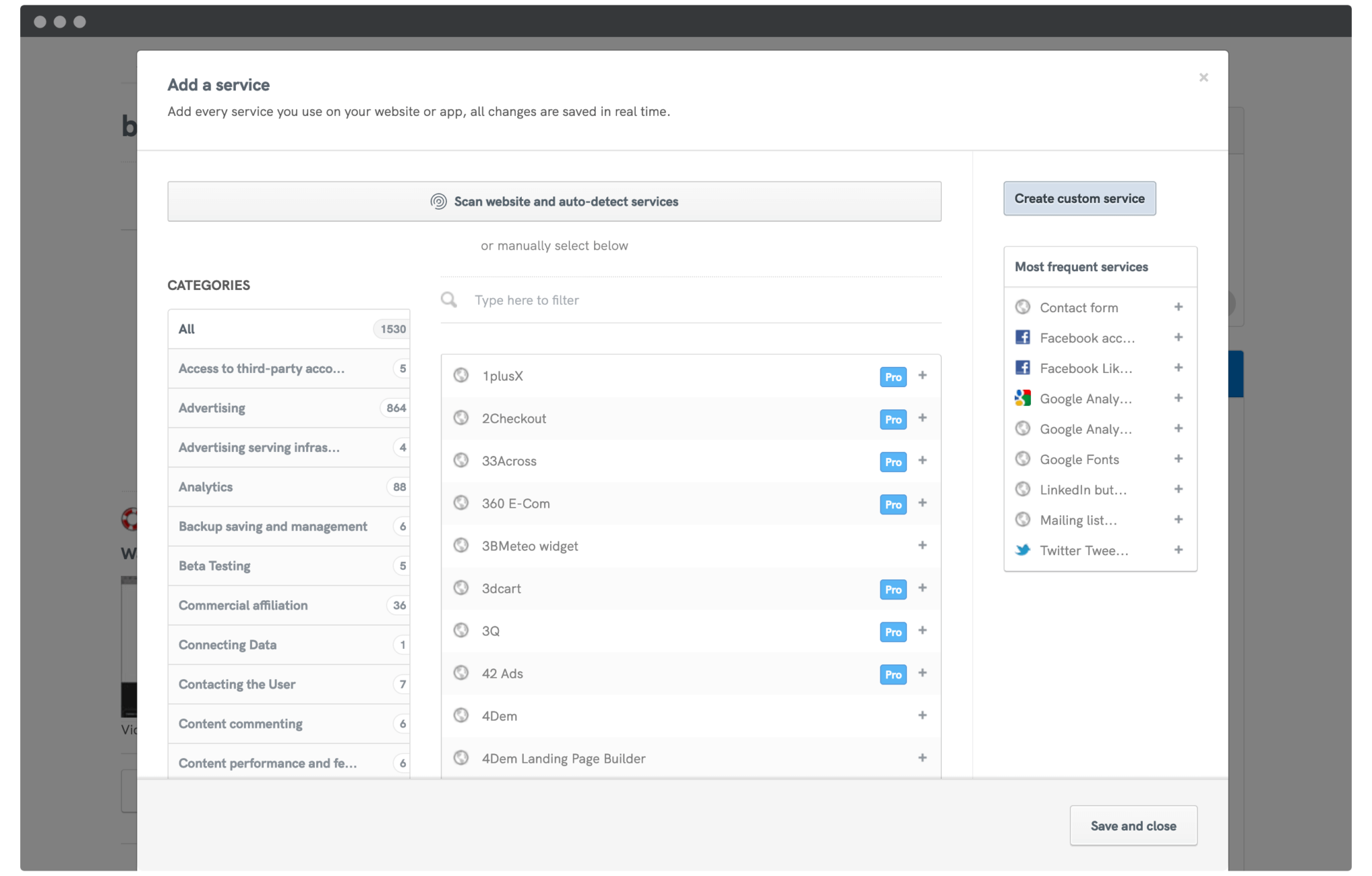Screenshot of a website displaying a user interface for adding services to a web platform or app. The headline reads "Add a Service," followed by a tagline instructing users to add every service they utilize. It emphasizes that all changes are saved in real-time. The website offers a feature to "Scan website and auto-detect services" and an option to "Create custom service." 

A list of frequently used services is displayed, including:
- Contact Form
- Facebook Account
- Facebook Like
- Google Analytics
- Google Fonts
- LinkedIn Button
- Mailing List
- Twitter Tweets
- T+X to Checkout
- 33 Across
- 36 Ecom
- 38 Metric Widget
- 3D Cart
- 3Q
- 42 Ads
- 4DEM
- 4DEM Landing Page Builder
- All 1,638 Services

There is detailed information about "Access to Third Party Account" categories, such as:
- Advertising (864 services)
- Advertising Serving Infrastructure (4 services)
- Backup and Management (6 services)
- Beta Testing (8 services)
- Commercial Affiliation (36 services)
- Connecting Data (1 service)
- Contacting the User (7 services)
- Content Commenting (6 services)
- Consent, Parker Performance (6 services)

This interface seems robust, offering a comprehensive list of integration options to enhance the functionality and tracking capabilities of a website or app.